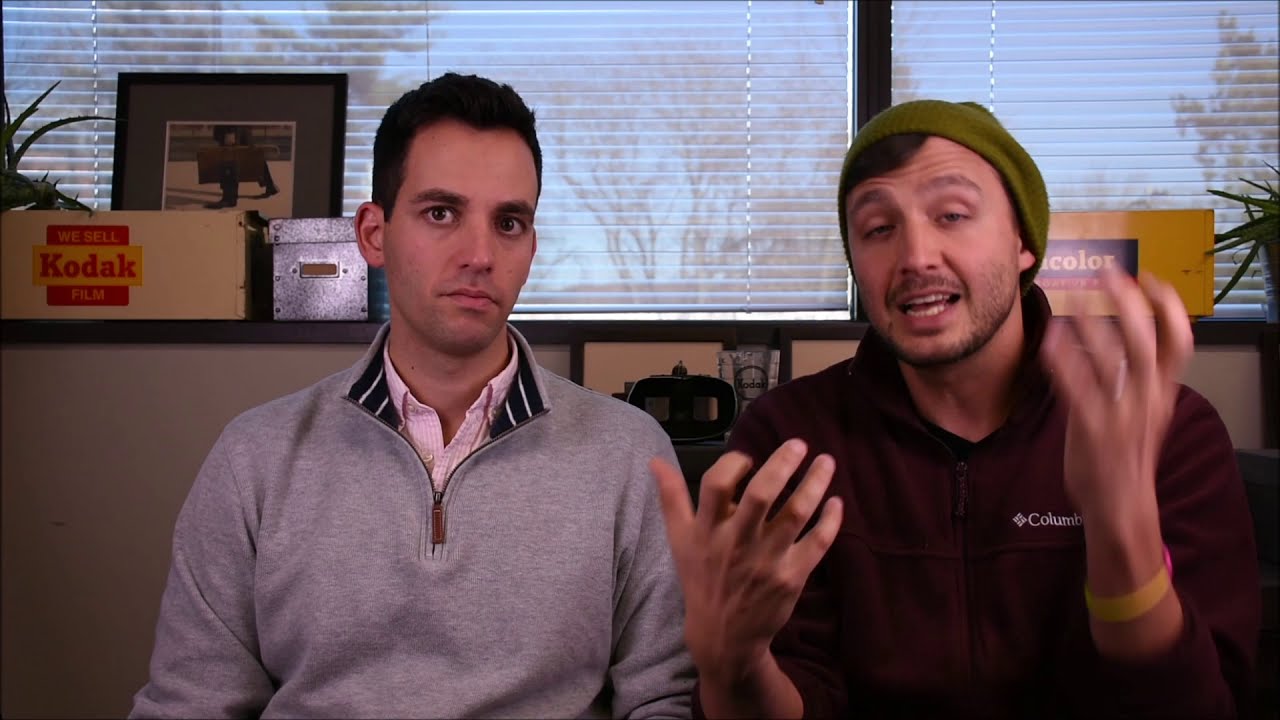This still image captures two Caucasian men in what seems like a paused video inside an office-like setting. The man on the right, who seems to be in mid-sentence, is wearing a green beanie and a burgundy hoodie with "Columbia" written on it. He has a light mustache and beard, and his raised hands are slightly blurred, indicating motion. The man to his left, dressed in a gray quarter-zip pullover over a pink collared shirt, gazes blankly ahead. Both appear to be young adults. Behind them is a white half-wall with brown framing, topped by windows adorned with partially translucent vertical blinds. Through the blinds, you can faintly see the sky, along with some bare and leafy trees. The windowsill in front contains various objects, including a photograph, a box labeled "Kodak," a silver box, and a couple of plants, suggesting a space associated with photography or media.